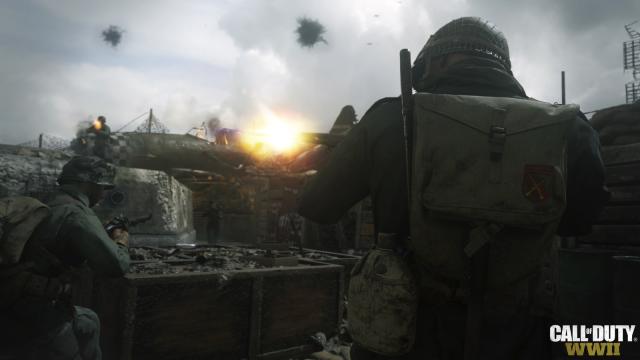The image, likely a screenshot from a video game called "Call of Duty: World War II," depicts a chaotic, war-torn battlefield. Dominating the foreground are two soldiers, one positioned on the left side and the other on the right. Both are dressed in traditional World War II military uniforms, complete with helmets, and are equipped with bags and firearms. They are actively engaged in combat, firing their weapons towards unseen targets in front of them, with vivid yellow and white flames erupting from the barrel of the gun held by the soldier on the right. Amidst the tumult, a wooden box provides scant cover for their advance. The backdrop reveals a grim scene with smoke clouds billowing into the sky from explosions, indicating ongoing aerial bombardments. In the far distance, one can spot a fighter plane, possibly a German aircraft from the war, its checkered front ablaze. Other soldiers can also be seen strategizing and firing, adding to the intensity of the scene. The bottom right corner of the image is marked with the game's logo, "Call of Duty: WWII," identifying it clearly as part of this well-known series of shooter-type war games.